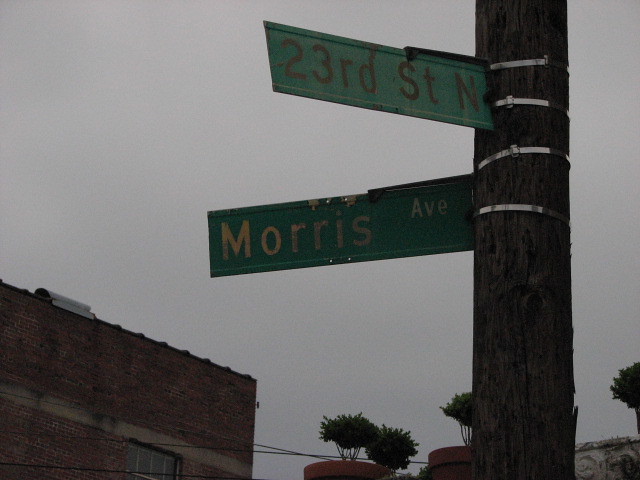This photograph captures an outdoor scene with the focus on a weathered brown utility pole, cocooned in decaying wood. The pole, stabilized by four silver zip ties, prominently displays two street signs. At the top, a gray sign reads "23rd Street North," and directly below it, an even grayer sign pointing to the left indicates "Morris Avenue." The image, though of low quality and enveloped in darkness possibly hinting at the onset of night, reveals a dark gray sky as its backdrop. In the lower left corner, the brick facade of a building emerges, while the lower right corner is occupied by the soft silhouettes of treetops.